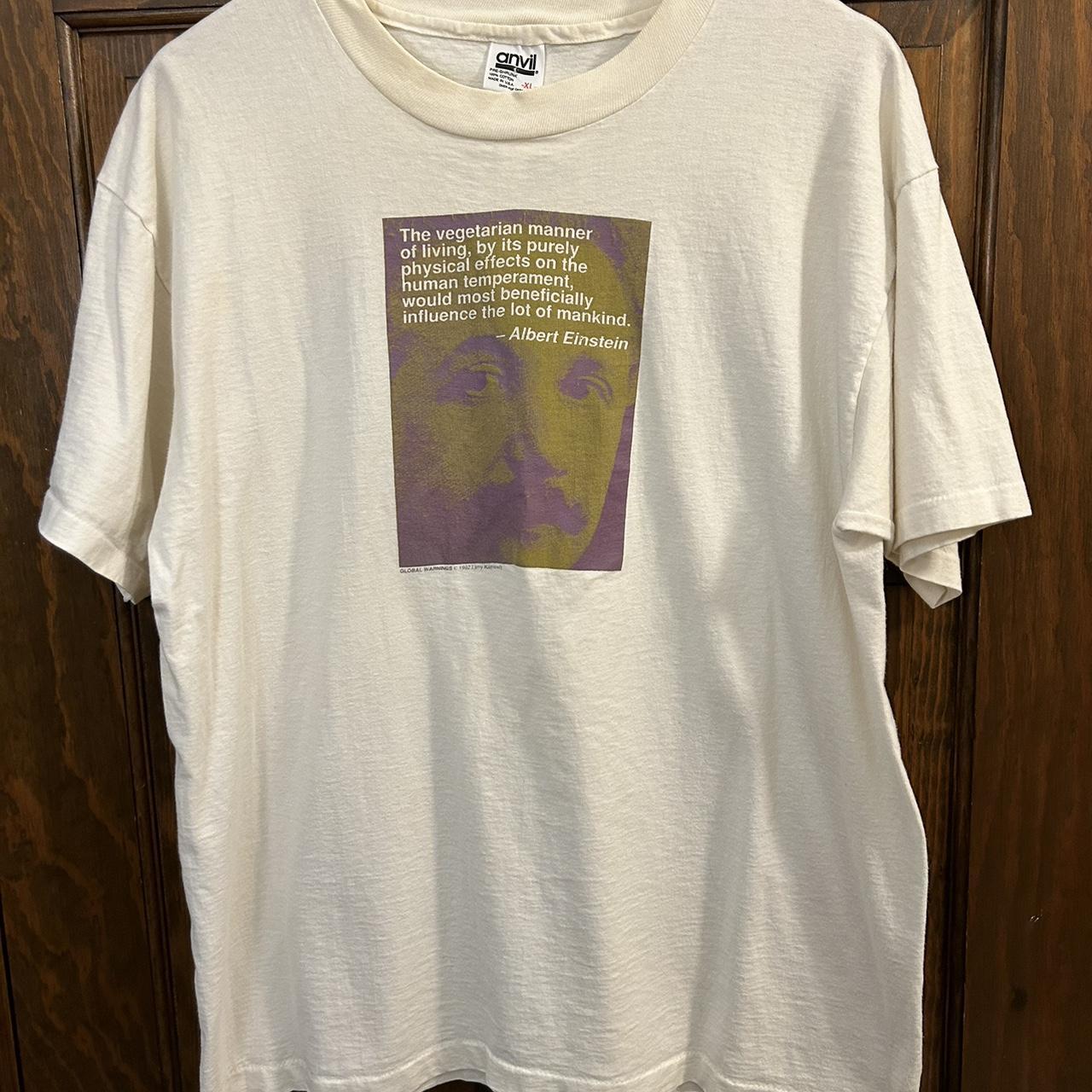The image depicts a well-worn white t-shirt hanging against a dark brown, possibly mahogany, wooden door. The door's vertical grain is clearly visible, contributing a rustic background to the scene. The t-shirt features a sepia-toned graphic of Albert Einstein in the center, accompanied by one of his quotes: "The vegetarian manner of living, by its purely physical effects on the human temperament, would most beneficially influence the lot of mankind. Albert Einstein." The shirt, identified as an Anvil brand by the visible inside tag, shows signs of extensive wear, particularly around the neckline, which appears dingy and in need of laundering. This suggests the shirt has been loved and worn frequently.